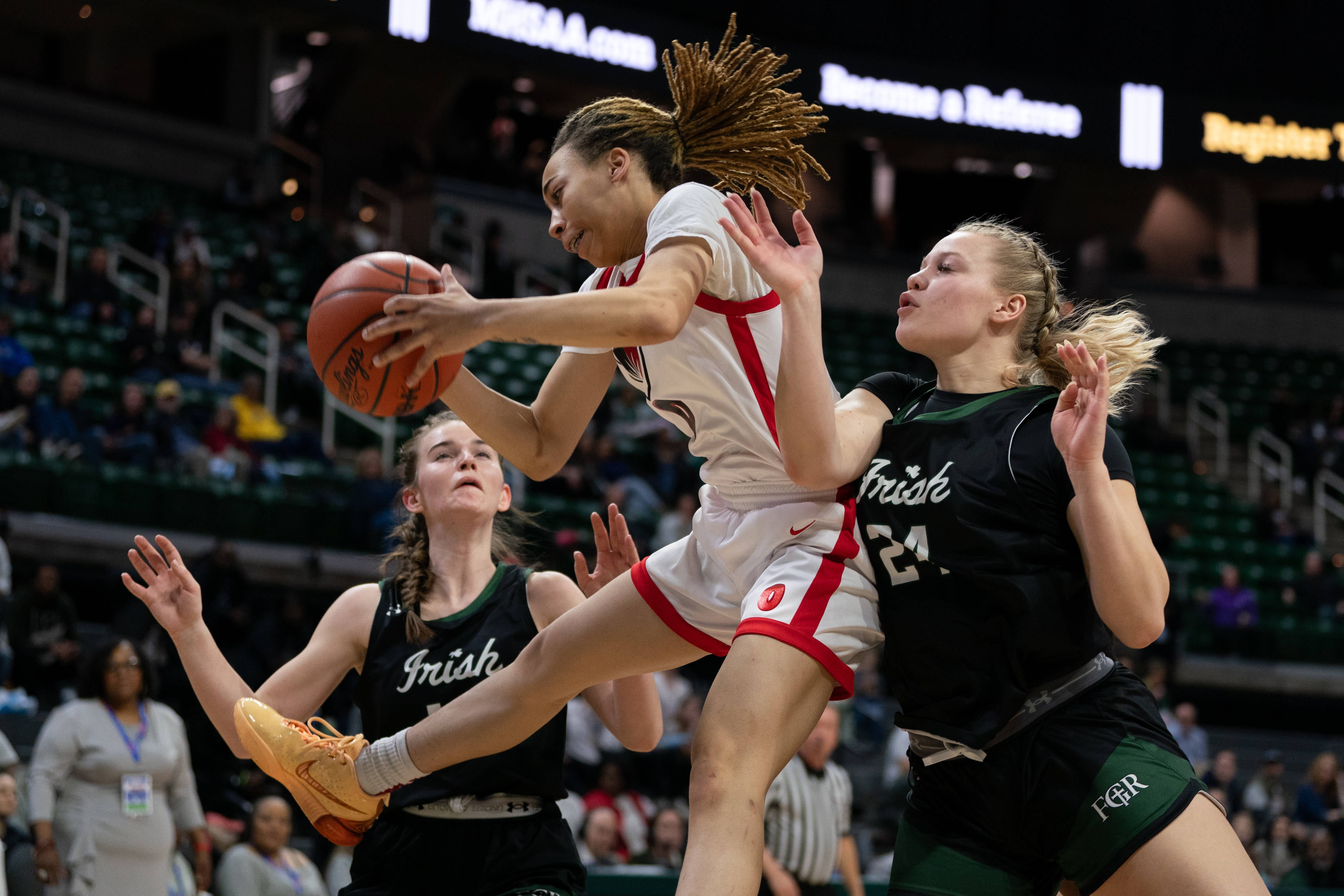In this dynamic image of a women's basketball game, the scene captures the intensity of the action from an upward perspective, focusing on three players. On the right, a player wearing a predominantly black jersey with green accents is prominently featured; her jersey displays the number 21 and a cursive inscription in white. Her shorts, matching in black and green, display the initials "FGR" with a cross intricately placed inside the letter "G." She has blonde hair and her arms are slightly raised as she participates in the play.

At the center, another player clad in a white and red jersey and sporting an orange Nike shoe leaps into the air, gripping the basketball with determination. Her long brown hair flows behind her, capturing the momentum of the jump.

To the left, a player in another black and green jersey appears with a perplexed expression and her hands raised in a questioning manner. 

In the background, the audience is visible, adding to the vibrant atmosphere of the game. Additionally, a coach stands at the bottom left corner, wearing a light gray long-sleeve shirt. She has black hair and is identifiable by a blue tag pinned to her shirt. This detailed snapshot encapsulates the energy and emotion of the game, highlighting both players and spectators alike.